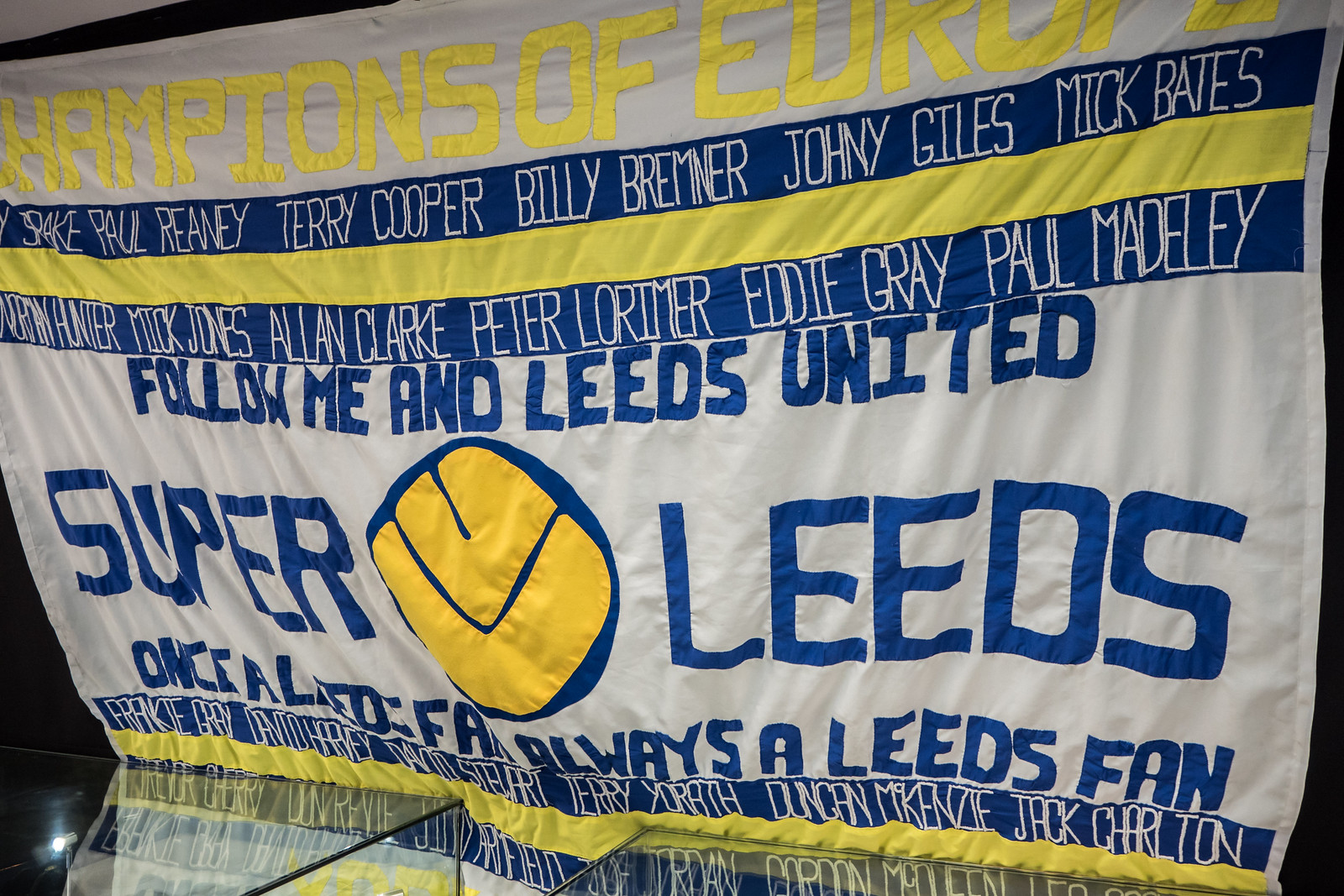This is a wide rectangular image of a large white fabric banner. The banner's text is prominently positioned slightly off-center at the top of the image, though partially cut off on the right side. At the top, bold, all-capital yellow sewn-on letters spell out "CHAMPIONS OF EUROPE." Below that, a blue rectangle displays in white font the names: "Paul Reaney, Terry Cooper, Billy Bremner, Johnny Giles, Mick Bates." There is then a yellow stripe followed by another blue stripe with additional names: "Mick Jones, Allan Clarke, Peter Lorimer, Eddie Gray, Paul Madeley." Beneath this, in bold blue letters, are the phrases "FOLLOW ME AND LEEDS UNITED," "SUPER LEEDS," and "ONCE A LEEDS FAN, ALWAYS A LEEDS FAN." The wrinkled banner makes some parts of the text difficult to read clearly, and there is a discernible yellow ball centered among the writings.